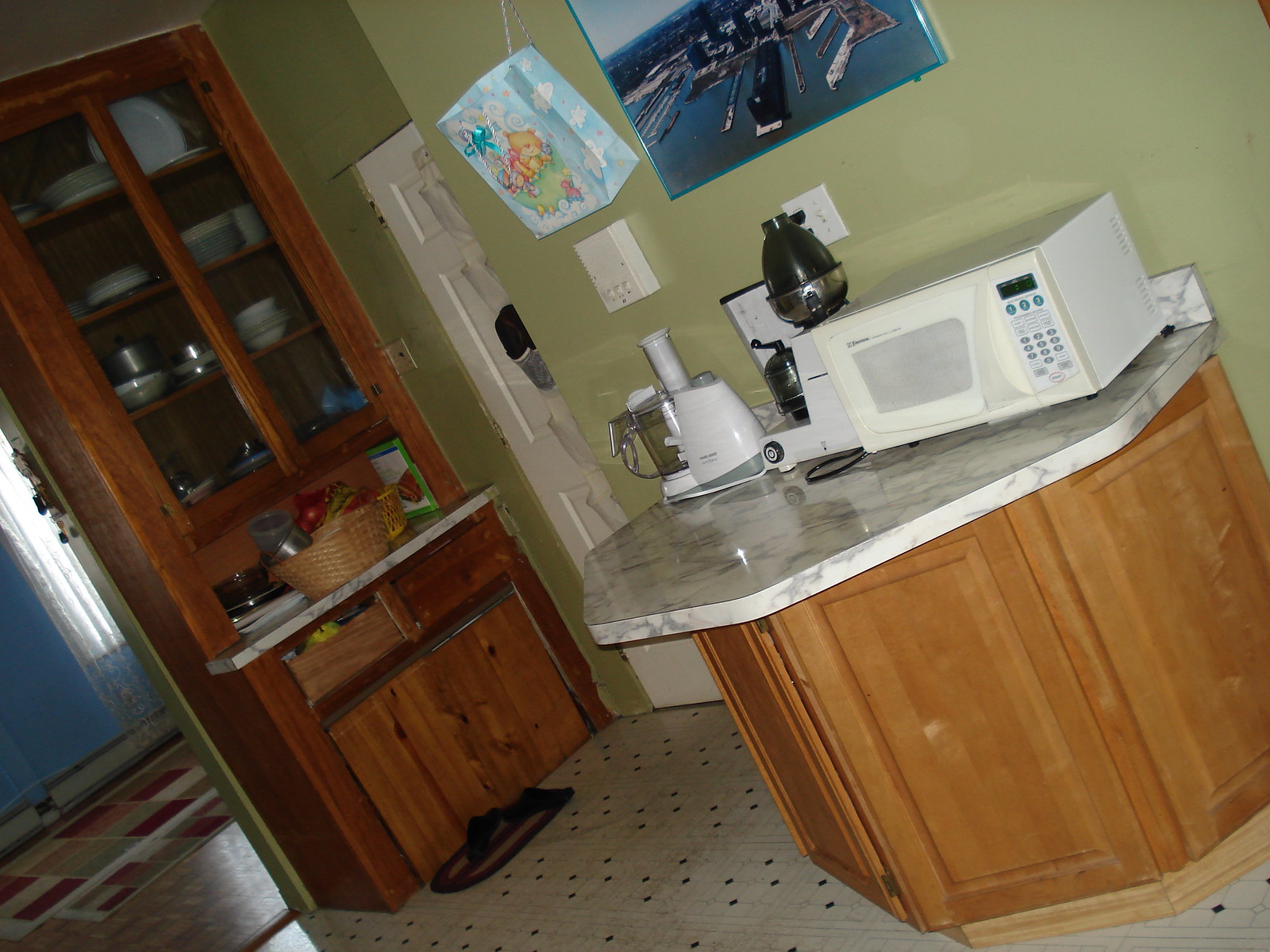The image depicts a kitchen from a right-angled, slightly slanted perspective. The central focus is an island that is attached to the wall, featuring wooden cabinets underneath. The countertop of the island boasts a sophisticated white and gray marbled design. Atop the island, there is a collection of white appliances, including a microwave, a coffee maker, and a food processor.

In the background, the wall is painted a light green color and adorned with a painting of a port scene with boats. To the left side of this wall is a light blue birthday gift bag. The wall continues back to reveal a white door. Adjacent to the door is another wall fitted with darker wood-colored cabinets that also feature the same gray and white marbling on the counter. These cabinets have transparent sections showing neatly arranged bowls and pots inside.

To the side of this cabinetry setup, an open wall area reveals the tile flooring, completing the scene of this organized and aesthetically pleasing kitchen space.